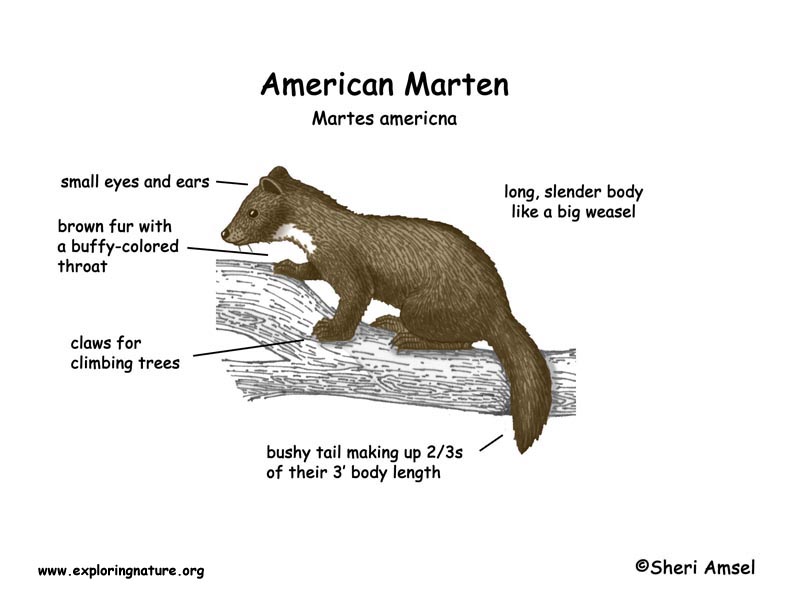The illustration depicts an American Martin, scientifically named Martes Americana, standing on a black and white drawn tree branch. This small, furry animal has predominantly brown fur, a buffy colored throat, and small eyes and ears. The Martin's medium-sized, bushy tail constitutes two-thirds of its three-foot body length. The detailed drawing includes labels with lines pointing to different body parts, such as "small eyes and ears," "claws for climbing trees," "long slender body like a big weasel," and "bushy tail." Positioned to the left, the Martin appears poised as if ready to move in that direction. The image, likely intended for educational purposes, possibly a children's book or interactive exhibit, includes credits reading "www.exploringnature.org" in the lower left and "copyright Sherry Amsel" in the lower right. The text is presented in black against the predominantly white background.